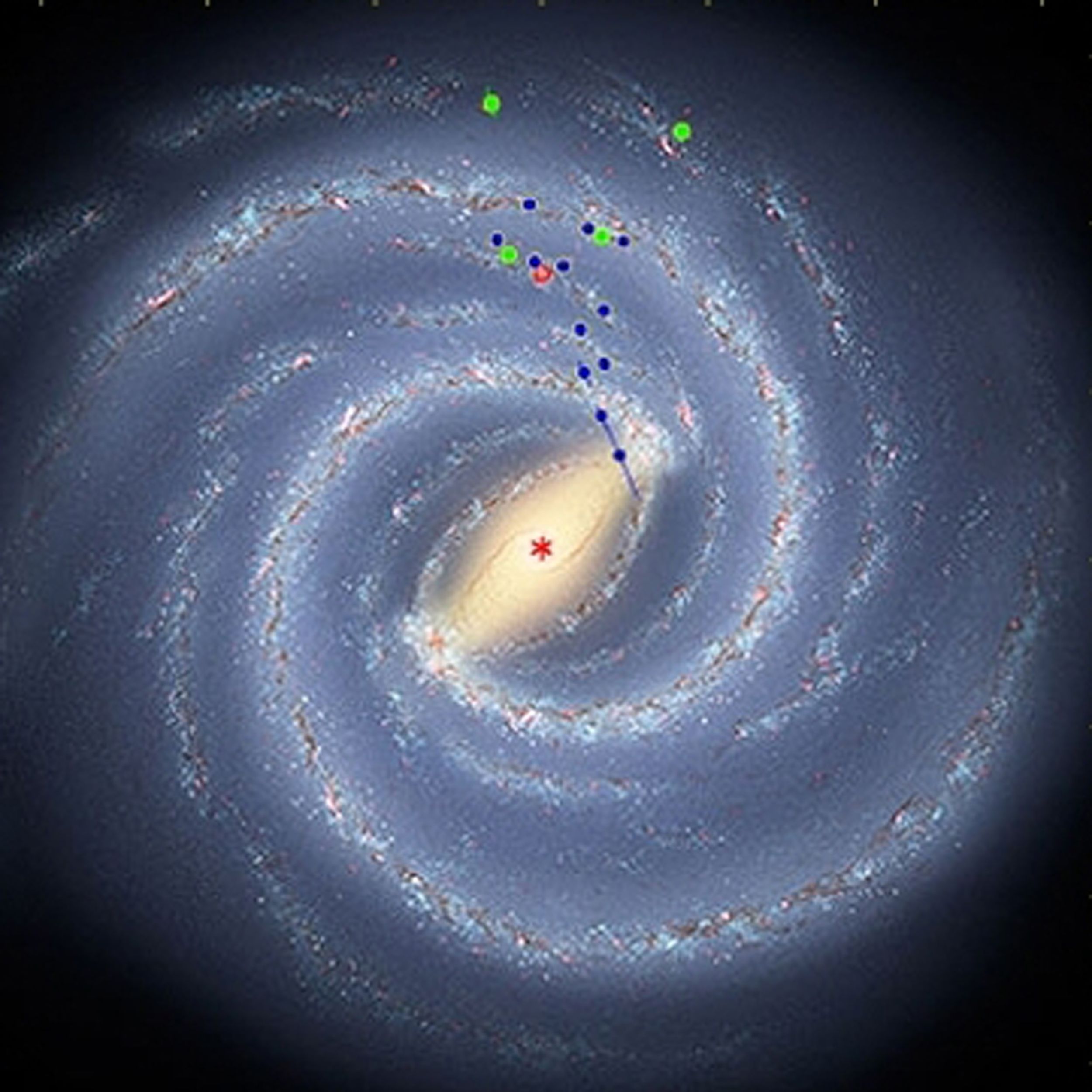The image portrays a vivid and possibly artistically enhanced galaxy, reminiscent of the Milky Way, with spiraling arms composed of stars creating a glittery or frosty appearance. The stars form round swirls rotating counterclockwise, centered around a radiant yellowish light with a small red asterisk-like star at its core. Scattered throughout the spiral arms are tiny, distinct blue and green dots. These dots appear meticulous, with some green ones touching while others remain isolated, and some blue ones connected by lines suggesting marked points of interest or annotation. The overall backdrop transitions to a deep black, enhancing the brilliance of the starry trails, with extra light giving a halo effect around the galaxy's arms. This image captures both the majestic awe of a galaxy and the detailed annotation typically seen in scientific imagery.